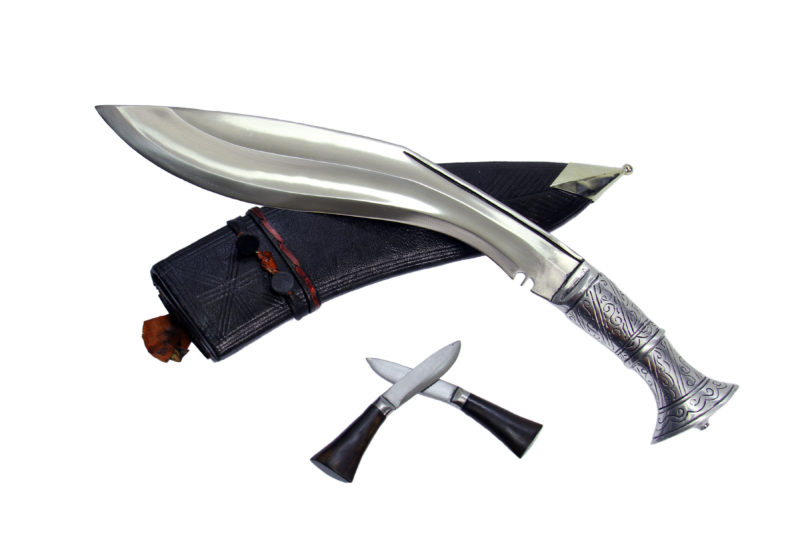The image depicts a collection of three distinct knives arranged against a plain white background. At the top is a prominently featured large knife resting on its sheath. The knife boasts a silver, ornate handle adorned with intricate swirl engravings and a shiny, slightly curved blade that widens towards the two-thirds mark from the handle. The black leather sheath beneath it has red decorative accents and a metallic tip to prevent the knife from piercing through. Below this set, two smaller knives are crossed in an X formation, with the left blade over the right. These small knives have black handles making up half of their length, connected by a silver band to their whitish blades. The composition creates a striking visual contrast between the elegant, detailed large knife and its sheath and the simpler, more utilitarian design of the smaller knives.